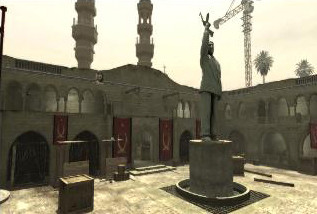The image depicts a deserted market square, seemingly from a computer game, dominated by a central statue of a figure with an arm raised in a manner reminiscent of a salute. The statue stands as a solitary sentinel amidst the empty space. In the background, a grand, castle-like building rises with its majestic archways and imposing structure. Draped on either side of the building are vibrant red tapestries, adding a splash of color against the stone facade. To the right, two tall trees stretch above the building, their presence adding a touch of nature to the otherwise stark and imposing scene.